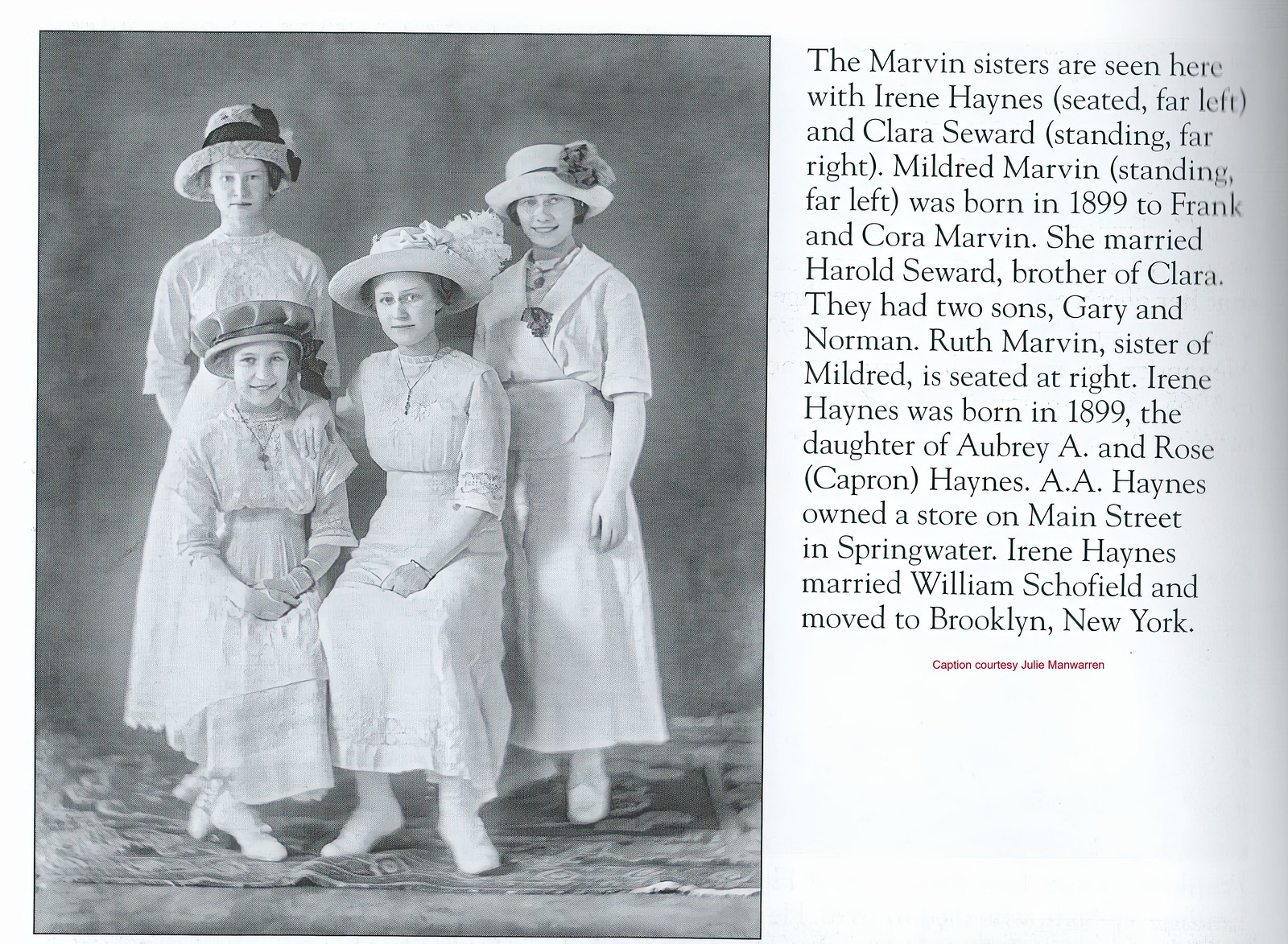The image is a wide, rectangular, black-and-white old-fashioned photograph on the left side of four women and girls dressed in turn-of-the-century clothing. Two women are seated in front with their hands folded in their laps, and two are standing behind them with their hands at their sides. All four wear elaborate wide-brimmed hats decorated with floral designs, ribbons, feathers, and some with black bands. Their white, lacy dresses reach their ankles, complemented by white stockings and slippers, presenting a unified, elegant appearance. The women are looking straight ahead, smiling, and appear joyful. On the right side of the image is a caption in black font that reads: "The Marvin sisters are seen here with Irene Haynes and Clara Seward. Seated far left is Irene Haynes, who was born in 1899 to Aubrey A. and Rose Catherine Haynes. Aubrey owned a store on Main Street in Springwater. Irene married William Schofield and moved to Brooklyn, New York. Standing far left is Mildred Marvin, born in 1899 to Frank and Cora Marvin, who married Harold Seward, brother of Clara, and had two sons, Gary and Norman. Clara Seward is standing far right, and Ruth Marvin, seated at right, is Mildred's sister."